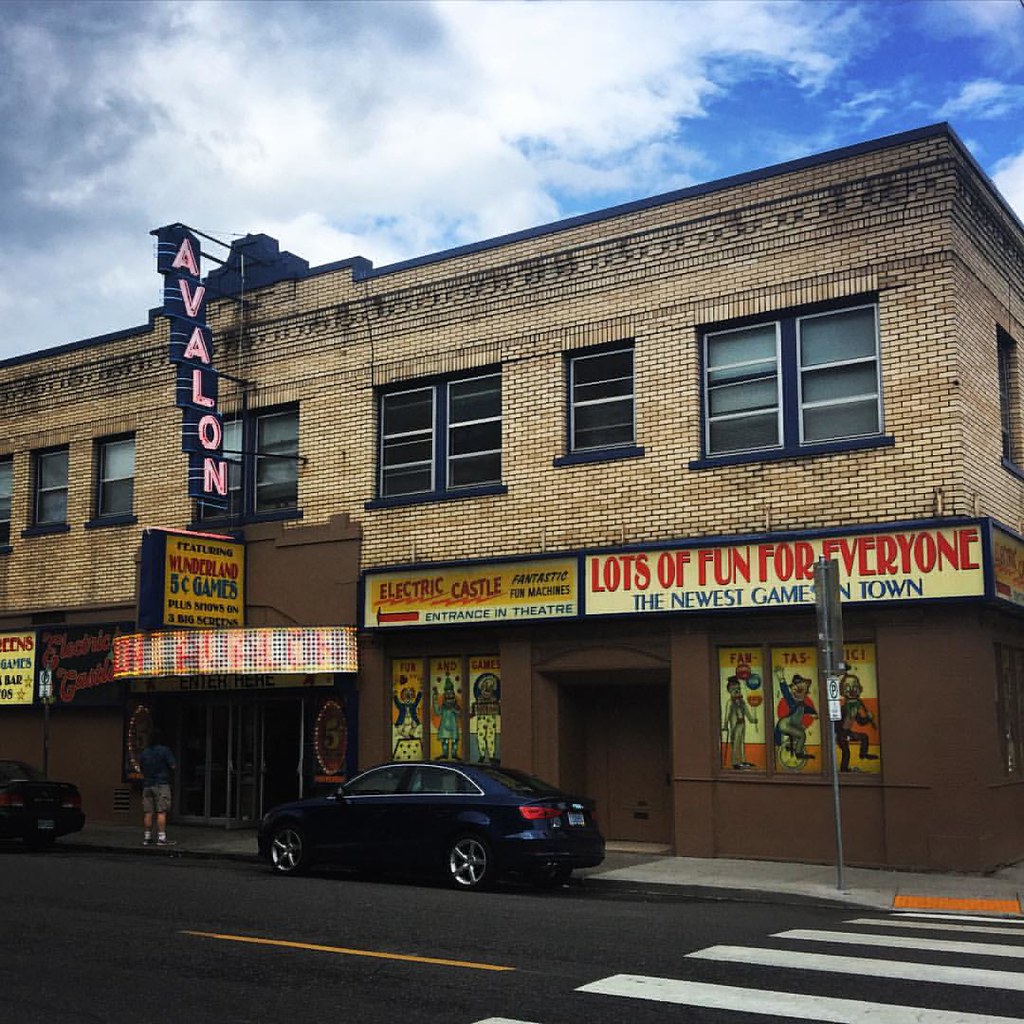This photograph captures the lively scene of an old downtown area featuring a prominent two-story brown brick building. The upper level showcases updated energy-efficient windows, some adorned with curtains while others remain dark. The building is fronted by a visually striking facade of multicolored bricks, adding an artistic touch. The focal point is a neon sign that reads "Avalon" in pink, positioned above the entrance to what appears to be an arcade or entertainment venue. Adjacent signs advertise "Electric Castle, fantastic fun machines, entrance in theater," and "Lots of fun for everyone, the newest games in town." Another sign highlights "Wonderland, five-cent games."

In front of the building, a man dressed in cargo shorts and a dark top stands near the entrance. Several posters, possibly featuring clowns, flank the doorway. Below, a black car is parked alongside the curb, and across the street, a dotted yellow line and crosswalk provide pedestrian access. The sky above features a mix of blue with clusters of gray and white clouds, completing this quaint yet dynamic cityscape.